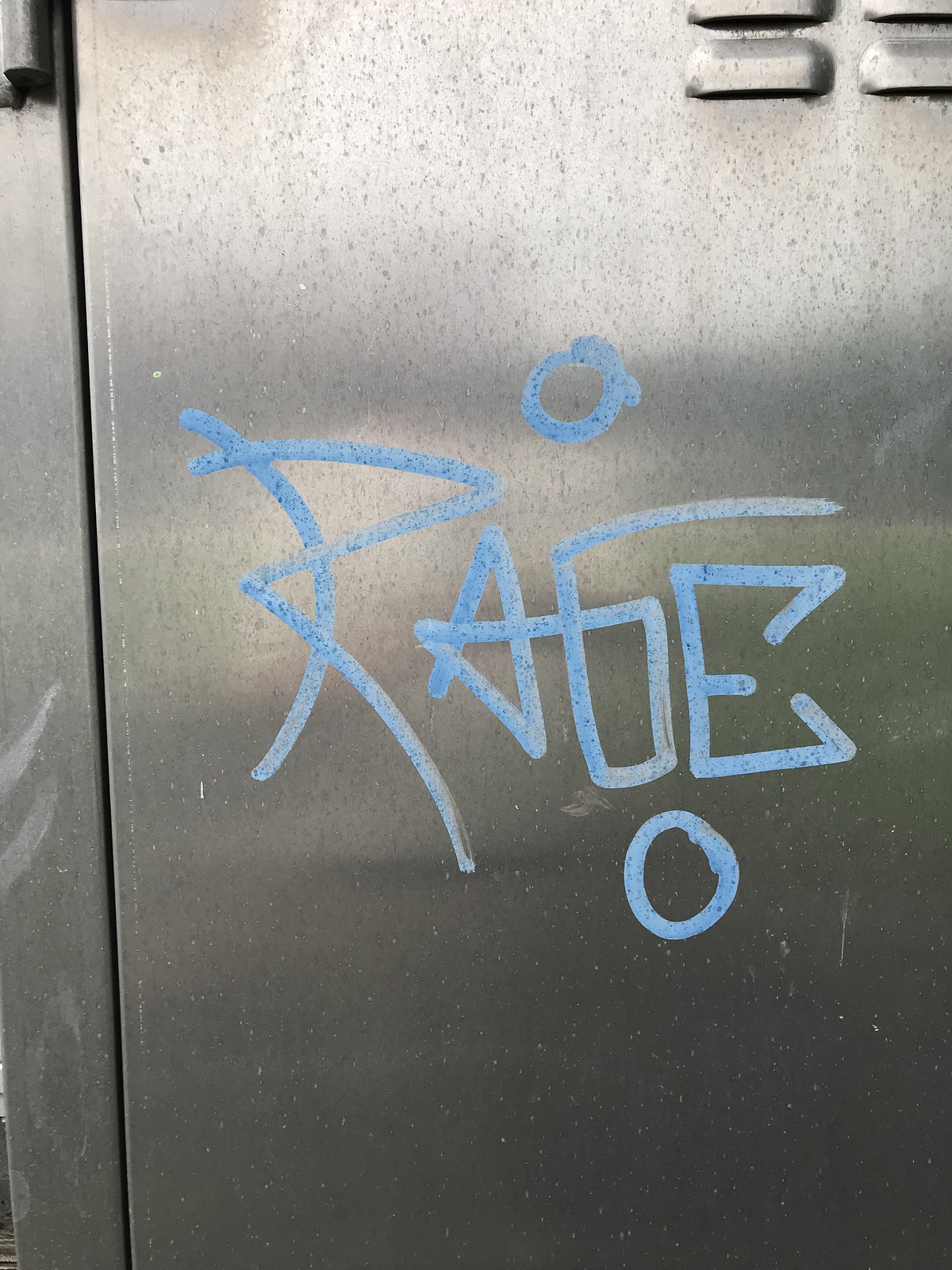This close-up image showcases the front of a metallic surface, likely a locker or a utility cabinet. The material appears to be stainless steel or aluminum, marked with spots possibly from rain or wear. The overall color of the surface is a silver-gray. In the upper right corner, there are a few air vents or louvers, while in the upper left, two black lines converge, adding to the utilitarian appearance.

The focal point of the image is graffiti rendered in light blue, either from a paint marker or brush. The graffiti spells out "RAGE" (R-A-G-E) with an exaggerated ornamental style, particularly on the letters "G" and "E." The complex design makes the "G" almost resemble a "B." Blue circles frame the word, one above and one below. The overall composition is devoid of people, focusing solely on the graffiti and the locker or cabinet.